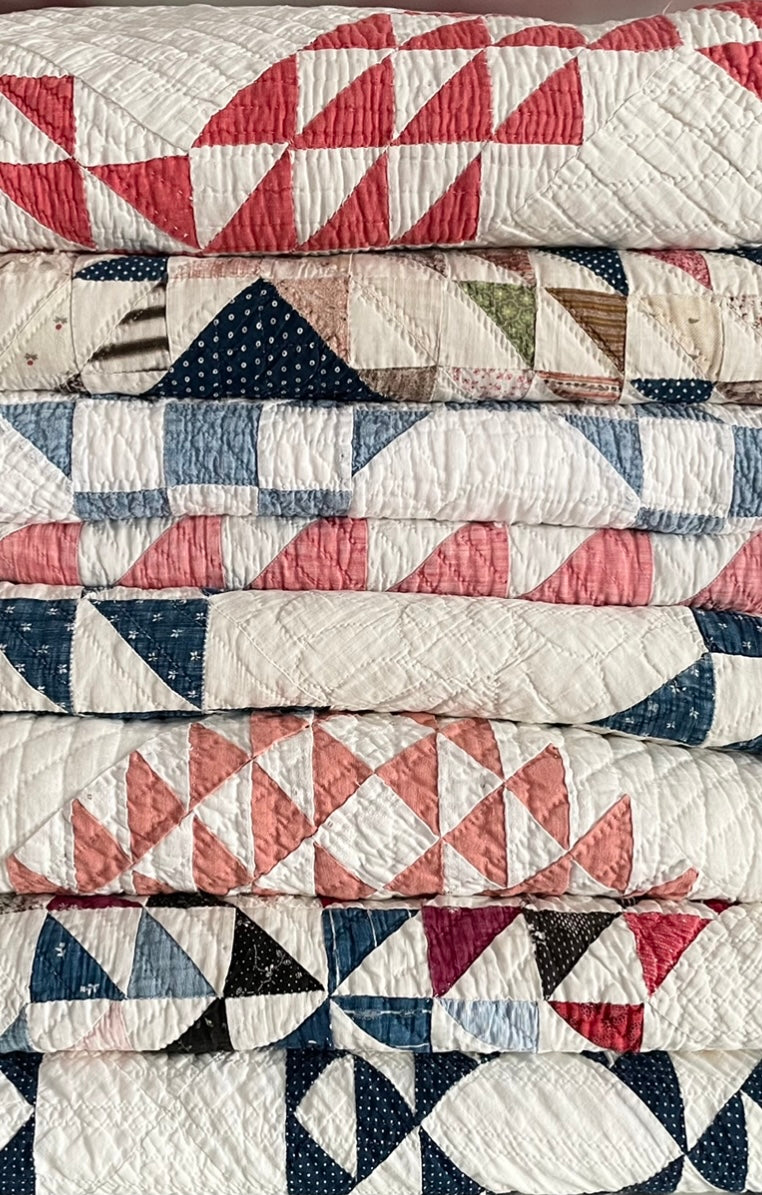The image features a collection of approximately eight rolled-up quilts neatly arranged side by side. Each quilt showcases a recurring geometric triangle pattern, where colored triangles—such as pink, red, blue, and dark peach—alternate with white triangles. The top quilt is predominantly beige and red, followed by a multicolored one with navy squares adorned with white dots, and patches in green, brown, and beige. Below these, a series of quilts display a variety of two-tone designs: a white and medium blue quilt, a dark pink and white quilt, a navy blue and white quilt, and a dark peach and white quilt. Another quilt prominently features patriotic red, white, and blue patches, while the bottom one is distinguished by white fabric interspersed with navy blue areas featuring white polka dots.